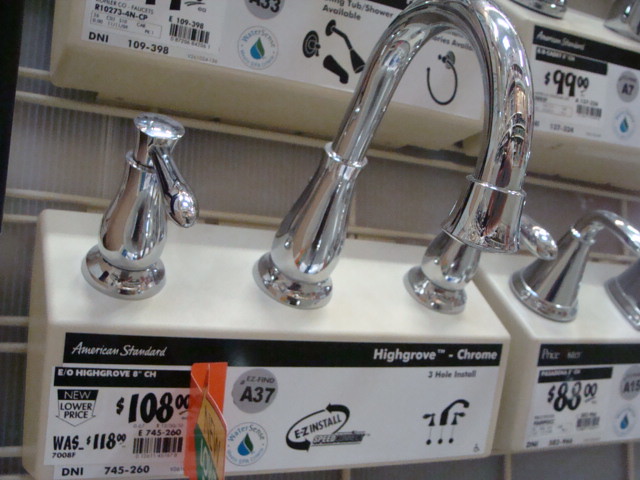This photograph, taken inside a store, showcases an up-close display of a chrome-colored bathroom faucet, most likely in a vanity or plumbing section. The central focus is an American Standard Highgrove Chrome faucet set, prominently priced at $108, reduced from its original $118, as indicated by the signage. The faucet, positioned in the center of the image, features a curved, swooping design, with the hot water handle on the left, the cold water handle on the right, and a sleek, shiny spout. Reflective surfaces capture the ambient lighting from the store, enhancing its polished appearance. The display is set against a corrugated wall with additional shelving where other models and price tags are partially visible, including another model priced at $88 and a tag showing $99. Placed below the faucet are detailed placards that provide product information, emphasizing its easy installation and stylish chrome finish suitable for modern bathroom decor.